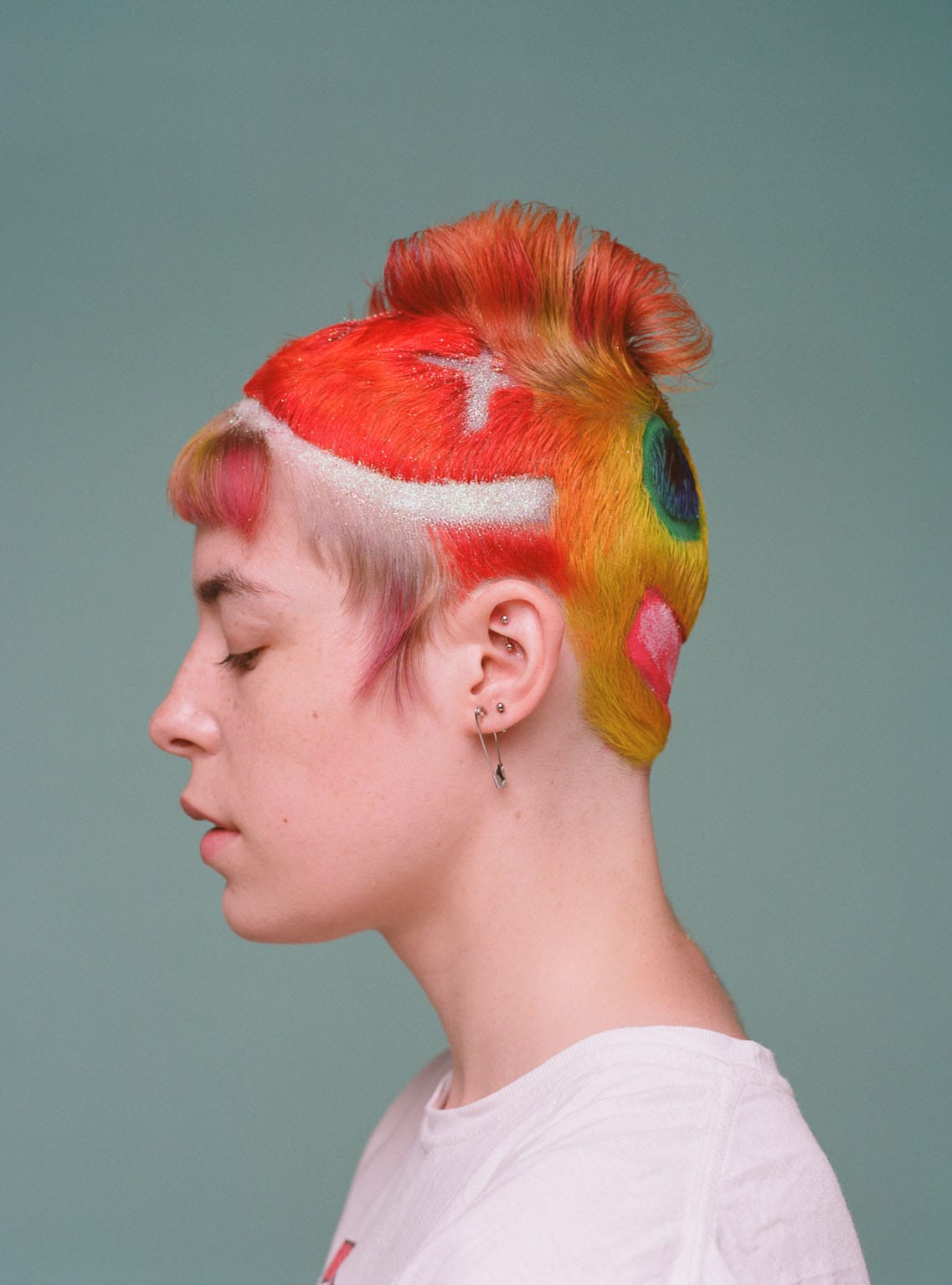The image is a vertically aligned, rectangular photo featuring a woman with a unique and vibrant hairstyle. She is shown in side profile, facing left, with her eyes closed and her mouth slightly open. Her hair is a striking mix of colors and styles: primarily reddish-pink and orange, with blonde and teal accents. She sports a mohawk-like cut with short hair at the back, dyed yellow with a smiley face, including green eyes and a pink mouth. There's also orange above her ear, and a cross-shaped shave on top with a loop of red and orange hair. Her bangs are a vivid mix of pink and yellow in the front. Several studs and a dangling earring adorn her ear. She wears a white t-shirt with something colorful on the front, although only her shoulders are visible. The background is a muted brown color, adding a subtle contrast to the overall vividness of her appearance.